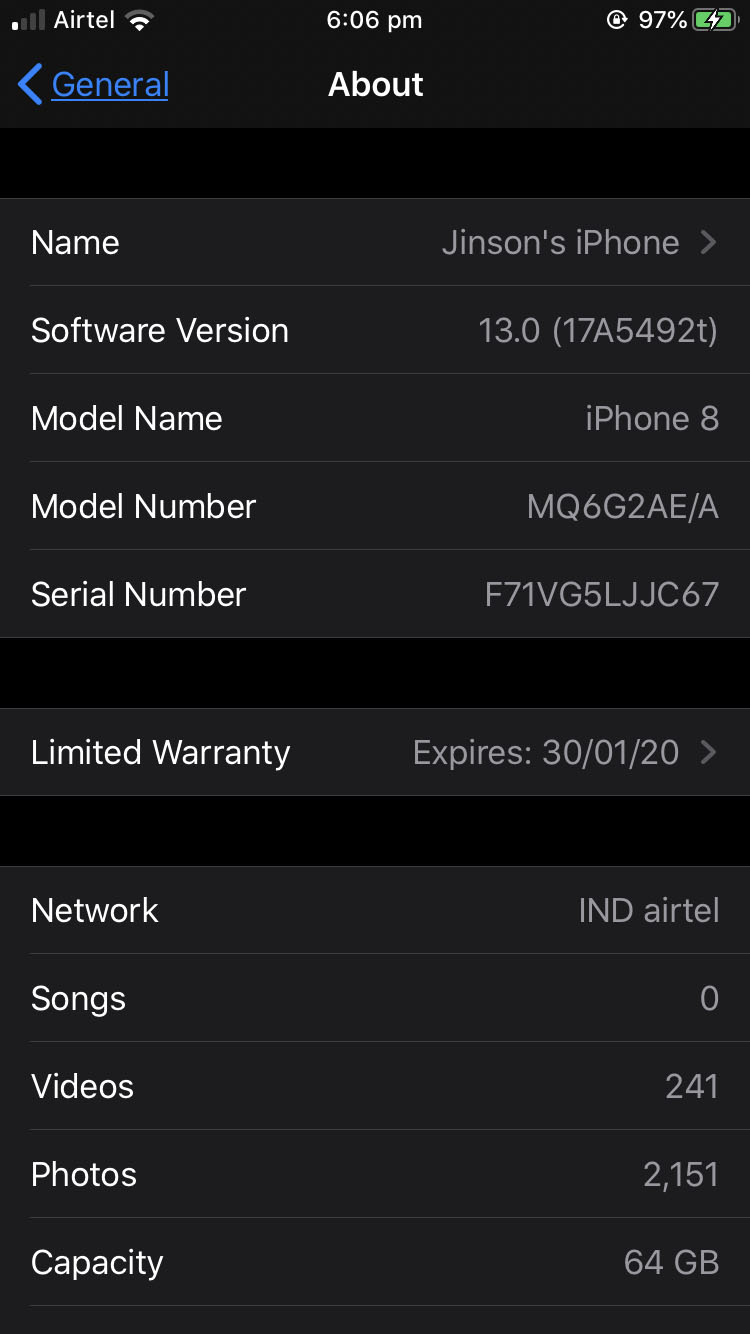A detailed caption for the described image:

"This image is a monochromatic screenshot featuring a summary of device information and status indicators for an iPhone 8. The backdrop predominantly displays shades of black and gray, indicating a minimalistic and professional user interface. At the top of the screenshot, 'Airtel' is indicated as the network provider, accompanied by a signal strength icon showing only one bar, denoting weak connectivity. The top-right corner displays the time, 6:06 p.m., along with a battery life indicator showing 97% charge remaining.

The main body of the screenshot comprises an 'About' section under 'General' settings which appears in darker black, creating a contrast with the adjoining interface elements. The 'Name,' listed as Jensen's phone,' and other technical details like the 'Software Version (13.0),' are presented in gray. Further details include the 'Model Name: iPhone 8' and some associated serial numbers, which are intentionally omitted.

A prominent dark black bar separates these details from the 'Limited Warranty' section, which is set to expire on January 30, 2020, indicating the information could be UK-specific due to the date format. Below the warranty information, additional device specifics are noted, such as the network provider 'IND, Airtel,' a tally of '0 songs,' '241 videos,' and '2,151 photos,' as well as the device's storage capacity, which is 64 gigabytes."